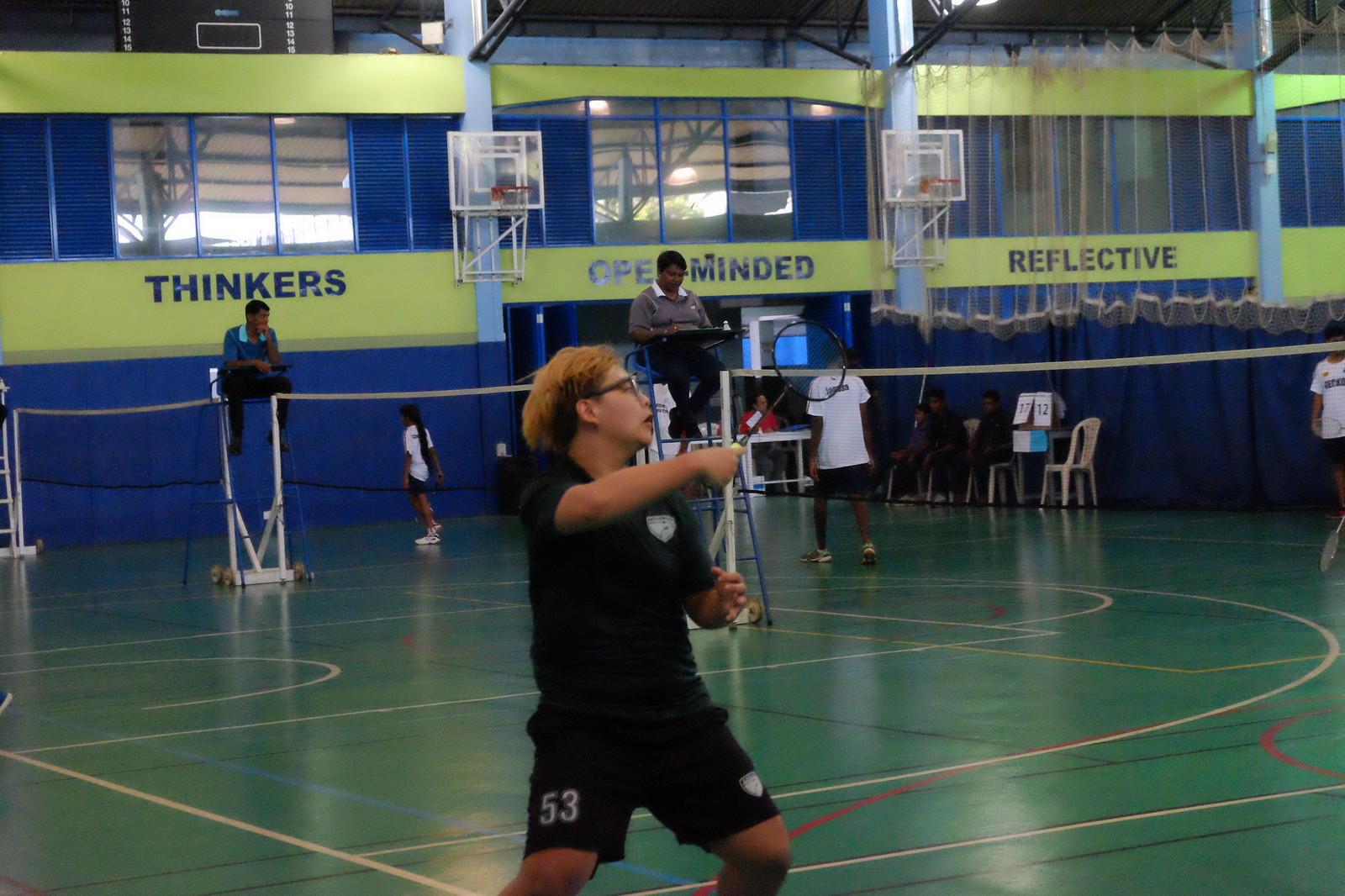In this detailed photograph taken inside a badminton indoor gymnasium, the central focus is a young boy with dyed red hair and glasses. He is wearing a black short-sleeved shirt and shorts, which appear to be a school uniform, with the number 53 prominently displayed on his shorts. He faces partly away from the camera, his face turned to the left, poised to swing a badminton racket with his right hand, likely in response to an incoming birdie. The gymnasium floor is predominantly green, intersected with various colored lines—white, red, blue, and black—indicating the boundaries for multiple games. A series of badminton nets frame the scene, with several participants visible beyond them. Notably, a girl wearing a white shirt and black shorts, along with other similarly dressed players, moves about in the background. Elevated seats house referees attired in gray collared shirts, diligently overseeing the matches. The gym's blue and yellow walls bear motivational words such as "thinkers," "open-minded," and "reflective," contributing to the inspiring ambiance of the space. Plastic lawn chairs scattered around host spectators and other participants, adding to the buzz of activity and competition within the gym. In the further background, two basketball goals are also visible, reinforcing the multipurpose nature of the facility.